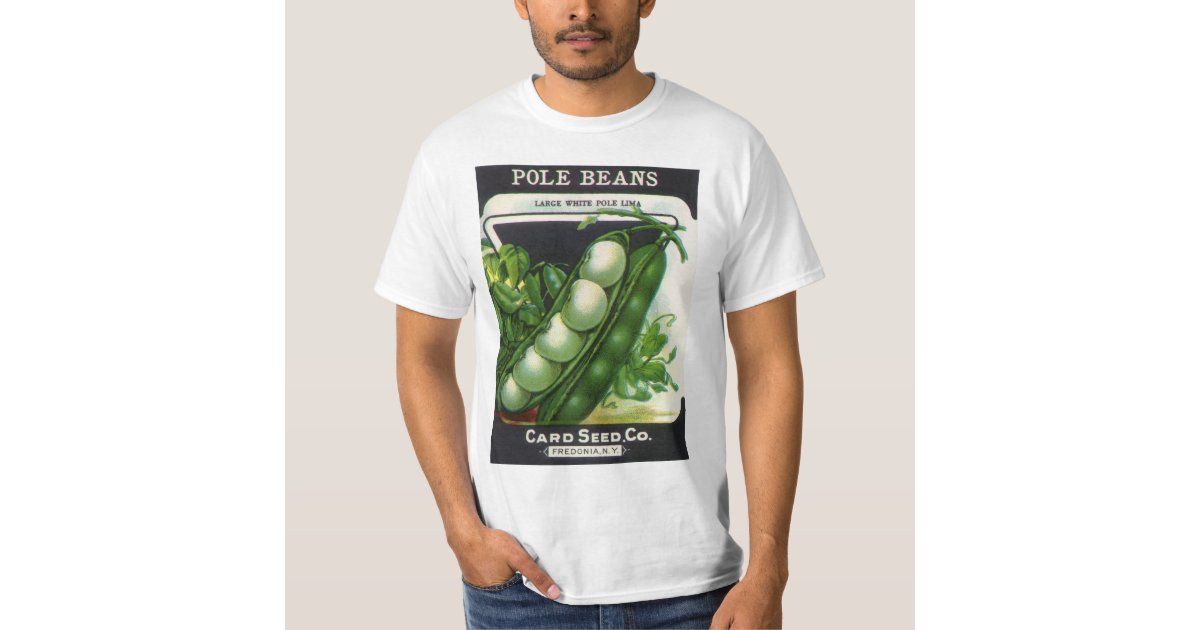The image features a medium to dark-skinned man with a shortly shaven beard, captured from his nose to the top part of his waist, set against a transparent or white background. He is wearing medium to dark blue denim jeans. His right hand is in his pocket with his thumb sticking out, while his left hand is out of his pocket. The man sports a white t-shirt adorned with a graphic design. The design includes a black banner at the top with the text "Pole Beans." Below this banner, it reads "Large White Pole Lima," and further down, "Card Seed Co. Fredonia York" is printed in black text on a white banner. The centerpiece of the t-shirt graphic features two peapods with visible peas inside, drawn in a mix of dark and lighter green hues, complemented by green leaves in the background.